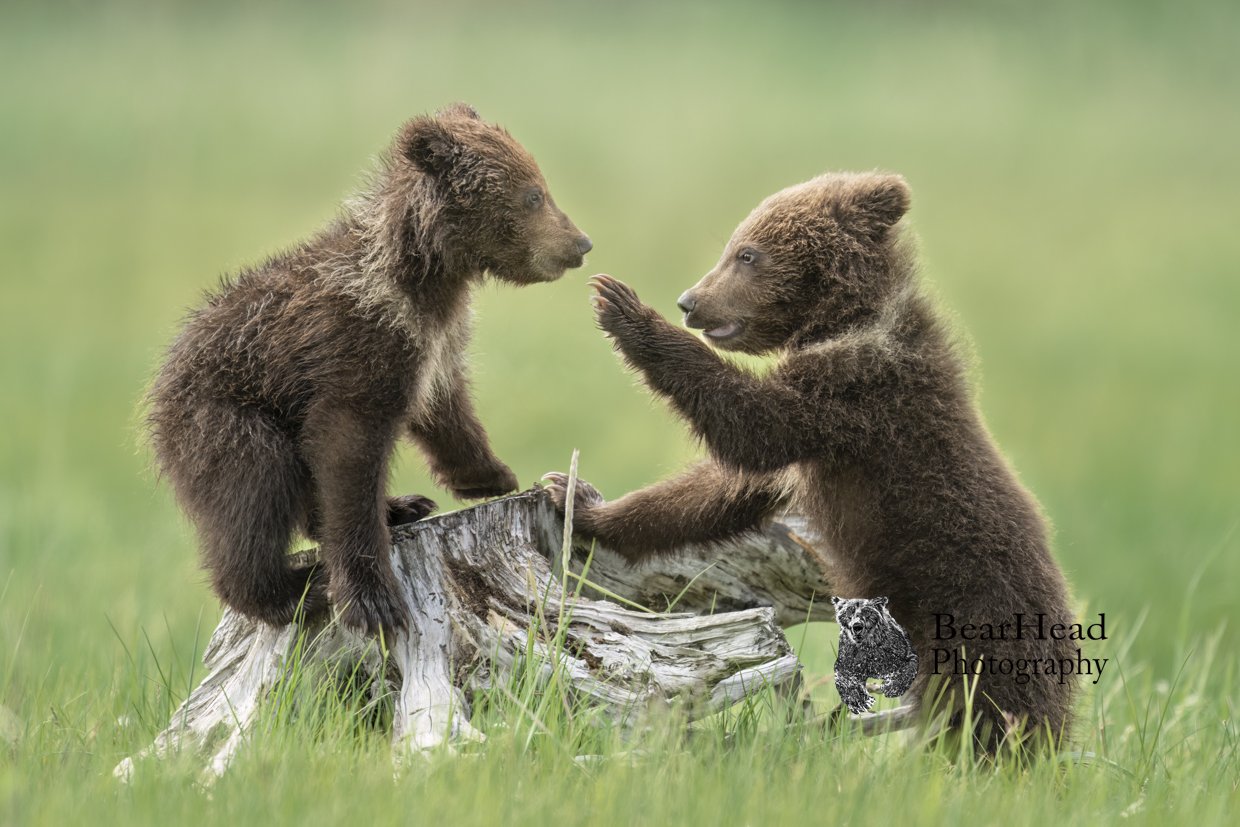The photograph, taken by Bear Lead Photography, depicts an enchanting scene of two playful brown bear cubs in a vibrant green field. The young bears, likely less than a year old, are captured in a moment of playful interaction near a tree stump. One cub stands on the stump, balanced on all four feet, facing its sibling, who is positioned on the ground with a raised front paw, engaging in a playful swipe. Their thick fur appears soft and insulating, ideal for their young age and any weather. The grassy field, which dominates the background, is artistically blurred, highlighting the natural, lively bond between the cubs. The image is bathed in natural light, enhancing the gentle, joyful essence of the moment. Additionally, the photograph features the Bear Lead Photography logo, an adult bear illustration, located in the right-hand corner, subtly framing this heartwarming display of youthful exuberance.